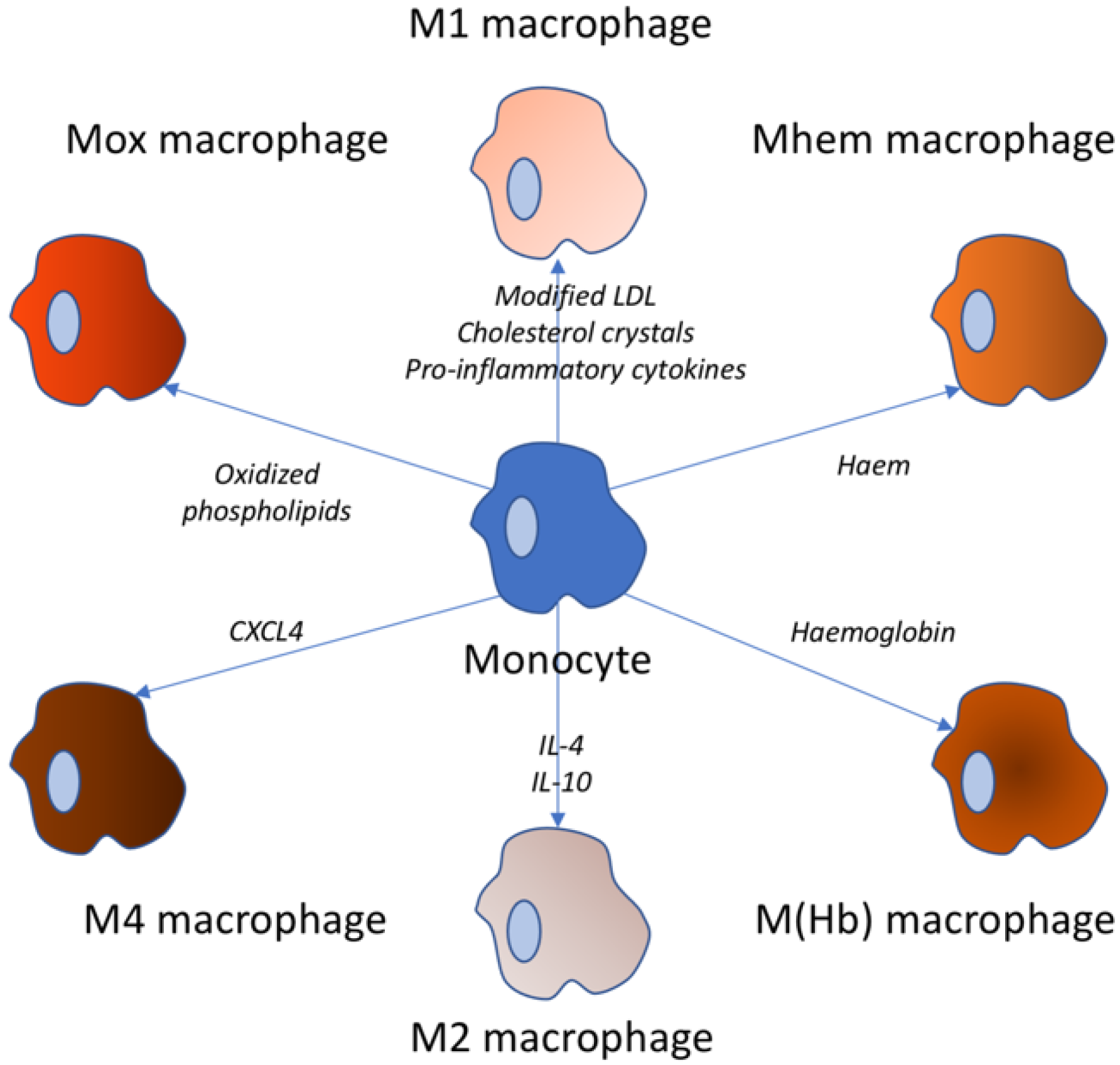This educational digital illustration features a detailed diagram of monocyte differentiation into various macrophages, set against a white background. At the center is a blue-colored monocyte, illustrated as a bluish blob. From this central monocyte, blue arrows radiate outwards to six different macrophages, forming a circular arrangement. Starting from the top and moving clockwise, the macrophages are labeled as follows: M1 Macrophage, MEM Macrophage, MHB Macrophage, M2 Macrophage, M4 Macrophage, and MOX Macrophage. Additionally, the image includes captions and labels for various stimuli and factors that influence this differentiation, such as modified LDL cholesterol crystals, pro-inflammatory cytokines, AIM oxidase, oxidized phospholipids, CXCL4, hemoglobin, IL-4, and IL-10. The title "M1 Macrophage" is prominently displayed at the top in black text, suggesting a focus on this specific type of macrophage within the broader context of monocyte transformation. The illustration serves as a comprehensive visual guide to the complex biological process of macrophage differentiation.